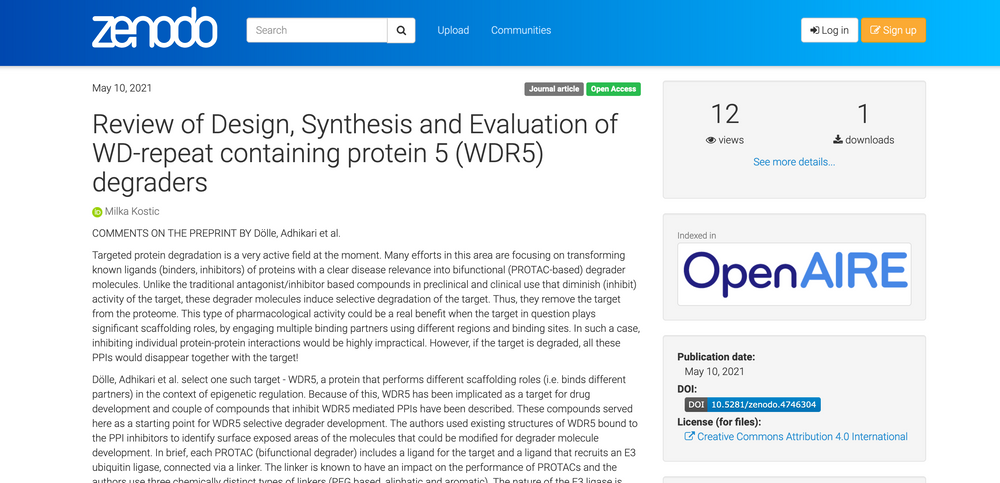A screenshot of a Zenodo webpage with a blue header prominently displaying the Zenodo logo on the left. To the right of the logo, there is a search bar, followed by links for "Upload" and "Communities." On the far right of the header, there are "Login" and an orange "Sign Up" button. The featured article, titled "Review of Design, Synthesis and Evaluation of WD Repeat Containing Protein 5 Degraders," authored by Milka Kostik, was published on May 10, 2021. Above the title, there are two tags: "Journal Article" and "Open Access." The visible portion of the article contains the first two paragraphs, but it likely extends beyond the screenshot. To the right of the article text, there are three informational boxes. The first indicates the article has 12 views and 1 download, with a link to see more details. The second box is an indexed ad banner for OpenAIRE. The third box lists the publication date (May 10, 2021) and the license (Creative Commons Attribution 4.0 International).